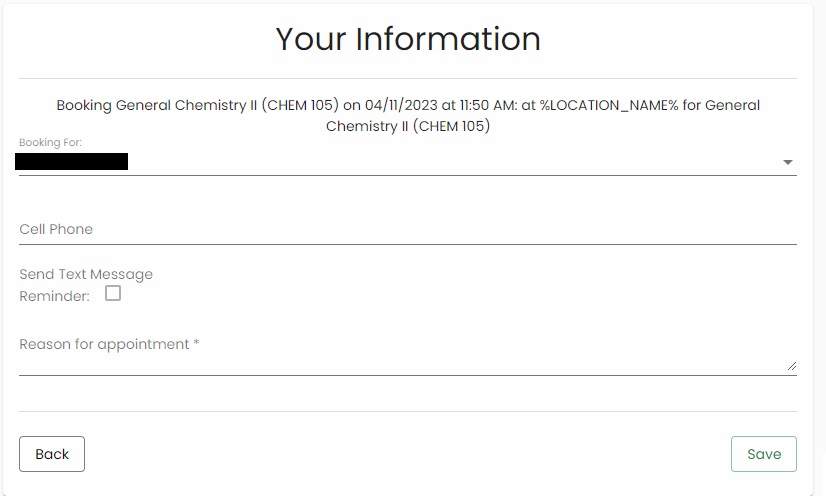At the center of the image, in black text, it states "Your Information." Directly beneath this, there's a heading: "Booking: General Chemistry 2" with the course code "(CHEM 105)" in uppercase and enclosed in parentheses. The specific booking date and time are noted as "4-11-2023 at 11:50 AM" at a placeholder labeled "Location – Name". This entire section appears to be a general appointment summary for a course booking.

Following this, "General Chemistry 2 (CHEM 105) Booking 4" is shown, with the surrounding text completely blacked out inside a square, obstructing any further details.

A long horizontal line stretches across the image. Above this line, there is a label that reads "Cell Phone" next to another label that says "Send Text Message Reminder" with a small, unchecked square box beside it.

Several inches below, a label "Reason for Appointment" is followed by a small asterisk, suggesting required information. An empty long line follows this label, possibly intended for user input but devoid of any existing text.

In the lower-left corner of the image, the word "Back" is enclosed in a square. In the lower right corner, approximately 8 inches away from "Back," the word "Save" is also enclosed in a square, indicating navigation or action buttons.